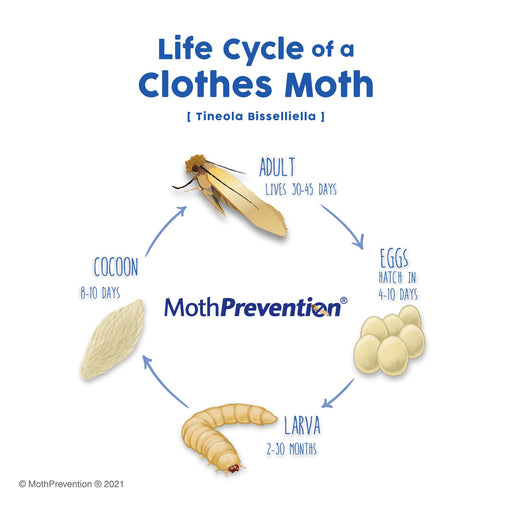This detailed image depicts the life cycle of a clothes moth (Tineola bisselliella) against a white background with all text in blue. At the top, it prominently reads "Life Cycle of a Clothes Moth," followed by the scientific name in smaller blue font underneath. The diagram is circular, made of arrows that progress through each stage of the moth's life cycle. 

Starting at the top, the first stage is labeled "Eggs" with the notation that they hatch in 4 to 10 days, accompanied by an image of the eggs. The arrow then moves downward to the "Larva" stage, depicted with an image of a small beige larva, and indicates that this stage lasts 2 to 30 months. Continuing upward, the next stage is the "Cocoon," shown with a whitish cocoon and annotated that it lasts 8 to 10 days. Finally, the arrows complete the cycle at the top with the "Adult" stage, illustrated by a brown-headed moth with a beige body and black legs, which lives for 30 to 45 days.

In the bottom left corner, there is a logo and a black copyright notice reading "Copyright Moth Prevention, Registered 2021." This detailed chart effectively outlines the sequential development stages of a clothes moth with clear visual and textual elements.